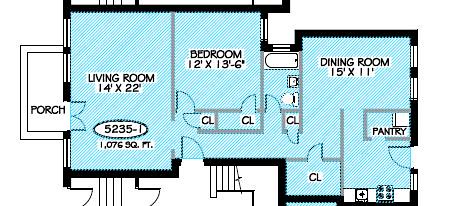This image features a meticulously designed online floor plan diagram outlined in black to illustrate the building's walls. Starting from the left side, the layout begins with a porch, indicated by a white rectangle labeled "porch." This area leads into a spacious living room measuring 14 feet by 22 feet, with all floors shaded in a light blue color for visual distinction.

From the living room, the plan progresses into a hallway that branches out to various rooms. To the right of this hallway is a bedroom measuring 12 feet by 13.5 feet, featuring two separate closet spaces within the hallway itself. Further down the hall, there is a combined bath and shower, a sink, and a toilet, as well as an adjacent closet accessible from this restroom area.

At the end of the hallway, there is an additional, slightly larger closet space. Directly across from this closet is the dining room, which seamlessly transitions into the kitchen area. The kitchen is equipped with a pantry located between the dining room and the kitchen space, providing ample storage.